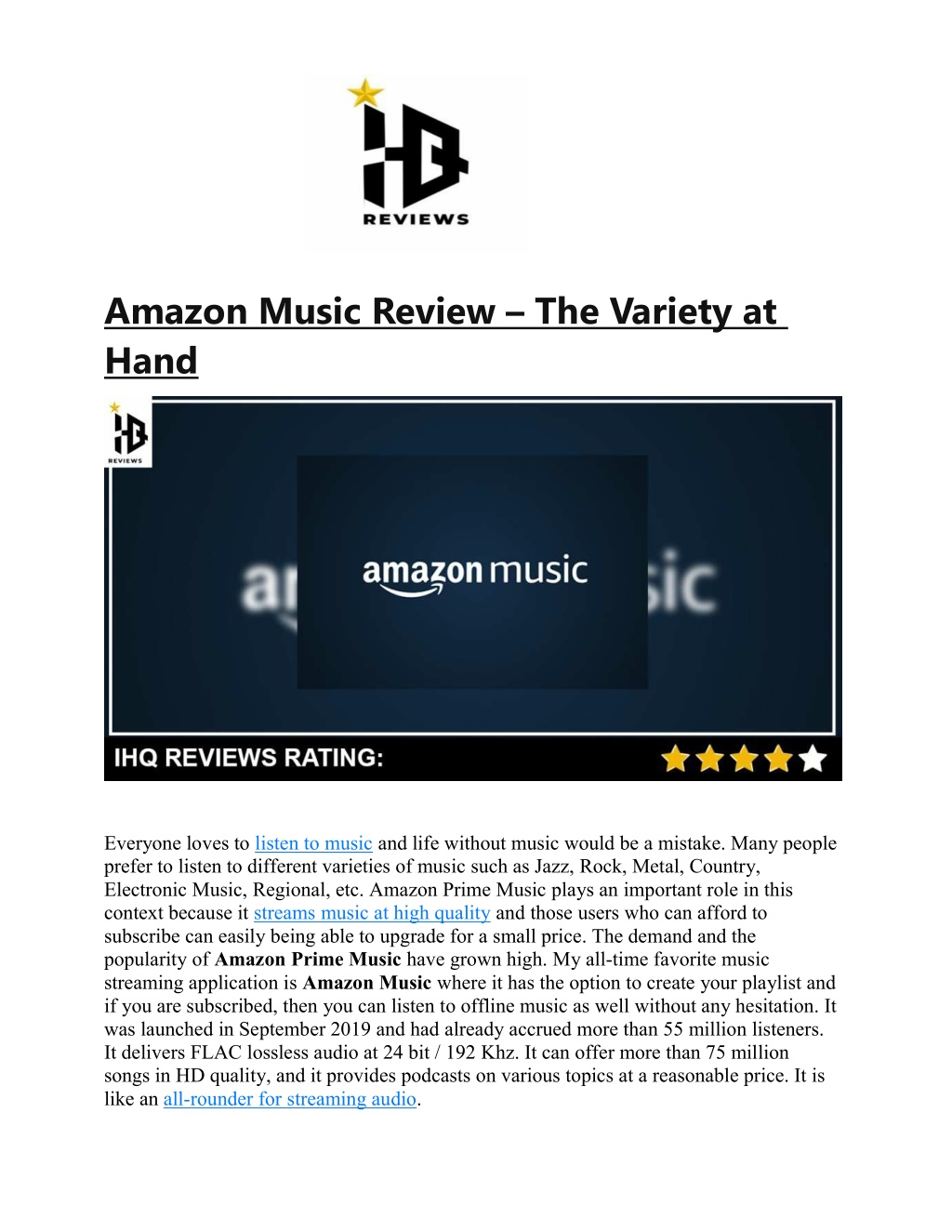The image features a detailed review of Amazon Music displayed on a screen. At the top, the word "Reviews" is prominently displayed, followed by a section titled "Amazon Music Review." Beneath this heading, there is an image displaying the words "Amazon Music" in white letters centered on the screen.

Below this, the image displays a rating box labeled "IHQ Rating" and "Reviews Rating," showing a score of 4 out of 5 stars, with 4 yellow stars highlighted and the fifth star remaining white. The review text starts with a hyperlinked statement, "Everyone loves to listen to music," continuing with the sentiment that "life without music would be a mistake." The review then elaborates on the different music genres people enjoy, such as jazz, rock, metal, country, electronic music, and regional music.

The review highlights the significance of Amazon Prime Music for high-quality music streaming, emphasizing that users willing to subscribe can upgrade their experience for a small fee. The text notes the increasing popularity and demand for Amazon Prime Music, with "Amazon Prime Music" and "Amazon Music" mentioned in bold black letters for emphasis.

The reviewer praises Amazon Music as their all-time favorite music streaming application, noting the option to create personalized playlists and access to offline music for subscribers. The review also mentions that Amazon Music was launched in September 2019 and has since gained over 55 million listeners. It offers FLAC lossless audio at 24-bit / 192 kHz and boasts a catalog of over 75 million songs available in HD quality. Additionally, the service provides podcasts on various topics at a reasonable price, describing it as an "all-rounder for streaming audio," which is hyperlinked in blue for further emphasis.